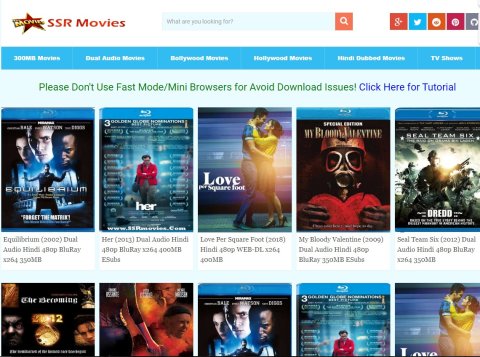A detailed caption for the image could be formulated as follows:

"The image depicts a website homepage dedicated to a vast collection of movies, identified as 'SSR Movies' prominently at the top. Adjacent to the title is a star icon also emblazoned with the word 'Movies'. Beneath the header, a search bar invites users to explore content with the prompt 'What are you looking for?' accompanied by an interactive orange magnifying glass icon. Positioned at the top are social media icons, including Twitter and other popular platforms, facilitating easy sharing and connectivity.

As you scroll down, the site organizes its offerings into sections starting with '300 MB Movies', 'Dubbed Movies', 'Hollywood Movies', a repeated 'Hollywood Movies' section, 'Hindi Dubbed Movies', and finally 'TV Shows'. A cautionary note in green text warns users, 'Please don't use fast mode/mini browsers for Android to avoid download issues,' paired with a clickable 'Click here for tutorial' link highlighted in blue.

The main content area showcases a streamlined list of movie options in rows of five. The first row features prominent titles: 'Equilibrium', 'Her', 'Love Per Square Foot', 'My Bloody Valentine', and 'Seal Team Six'. This pattern of presenting five movie options in successive rows continues down the page, offering users an extensive array of viewing choices."